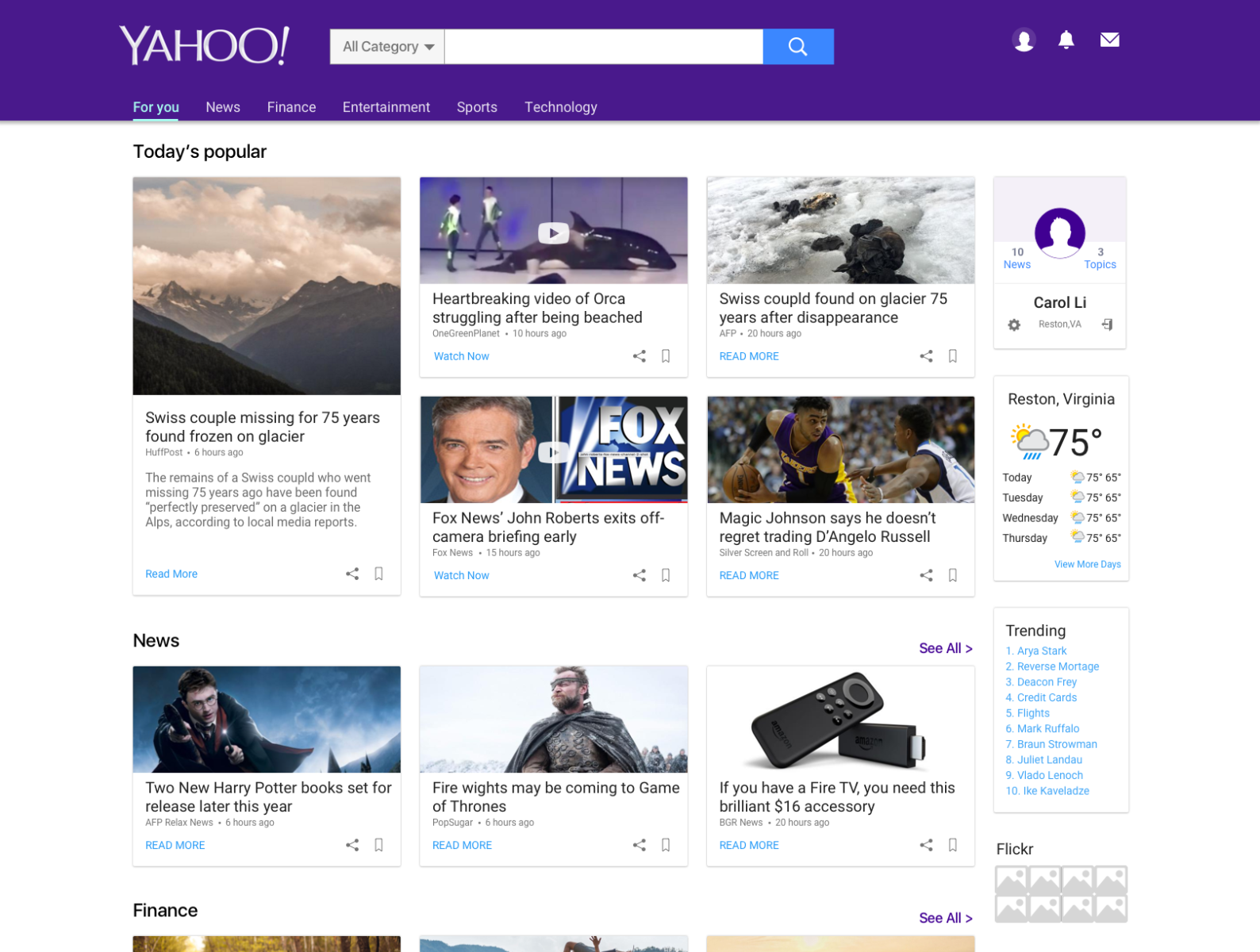Displayed on the screen is the Yahoo website, characterized by a prominent purple banner at the top and the word "Yahoo" in capital white letters. To the right of the Yahoo logo is a search bar with the placeholder text "All Categories," accompanied by a blue button for initiating the search. Currently, the search bar is empty.

To the right of the search bar, there are three icons: a user profile icon, a notifications icon, and a mail icon likely leading to the email inbox. Just below the banner is a navigation bar with several categories: "4U," "News," "Finance," "Entertainment," "Sports," and "Technology." The "4U" tab is currently selected, displaying its content.

On the "4U" page, under the section titled "Today's Popular," various articles are listed:

1. A headline about a Swiss couple found frozen 75 years after going missing on a glacier, which is highlighted as a tragic event.
2. An article featuring a heartbreaking video of an Orca struggling after being beached.
3. A repeat of the initial story about the Swiss couple found on the glacier.
4. A report on Fox News indicating that John Roberts briefly exited off-camera during a briefing.
5. An article where Magic Johnson discusses not regretting the trade of D'Angelo Russell.

To the right of these articles, there is a weather widget displaying the current conditions in Reston, Virginia, showing a temperature of 75°F with an image of clouds and rain. The widget also provides a forecast for the rest of the week.

Additionally, there is a section dedicated to trending topics, followed by more news articles. Overall, the page provides a comprehensive overview of trending news, personalized content, and current weather conditions.